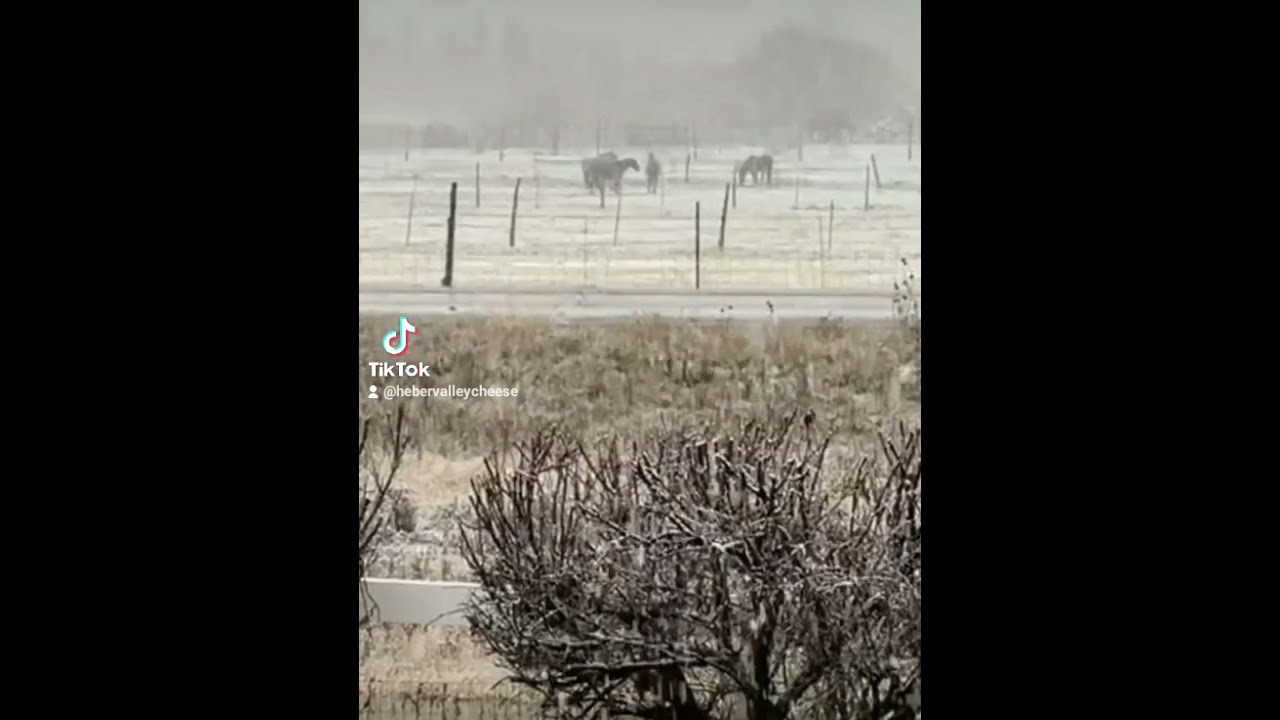This image is a screenshot from a TikTok video, captured vertically which results in black banners on either side. It prominently features an outdoor farm scene characterized by a variety of elements. In the foreground, there's a shrubbery tree and some light gray-green bushes below it. The middle ground contains three horses grazing with a man standing amongst them on a very light, off-yellowish field, giving the appearance of a winter day with a light dusting of snow. The background is dominated by a dusty light gray ambiance, contributing to the overall foggy and overcast atmosphere. The center of the image displays the TikTok logo along with the handle "@HeberValleyCheese." The image's edges feature black backgrounds, enhancing the contrast of the central farm scene and emphasizing the pastoral tranquility of the setting despite the gloomy weather.